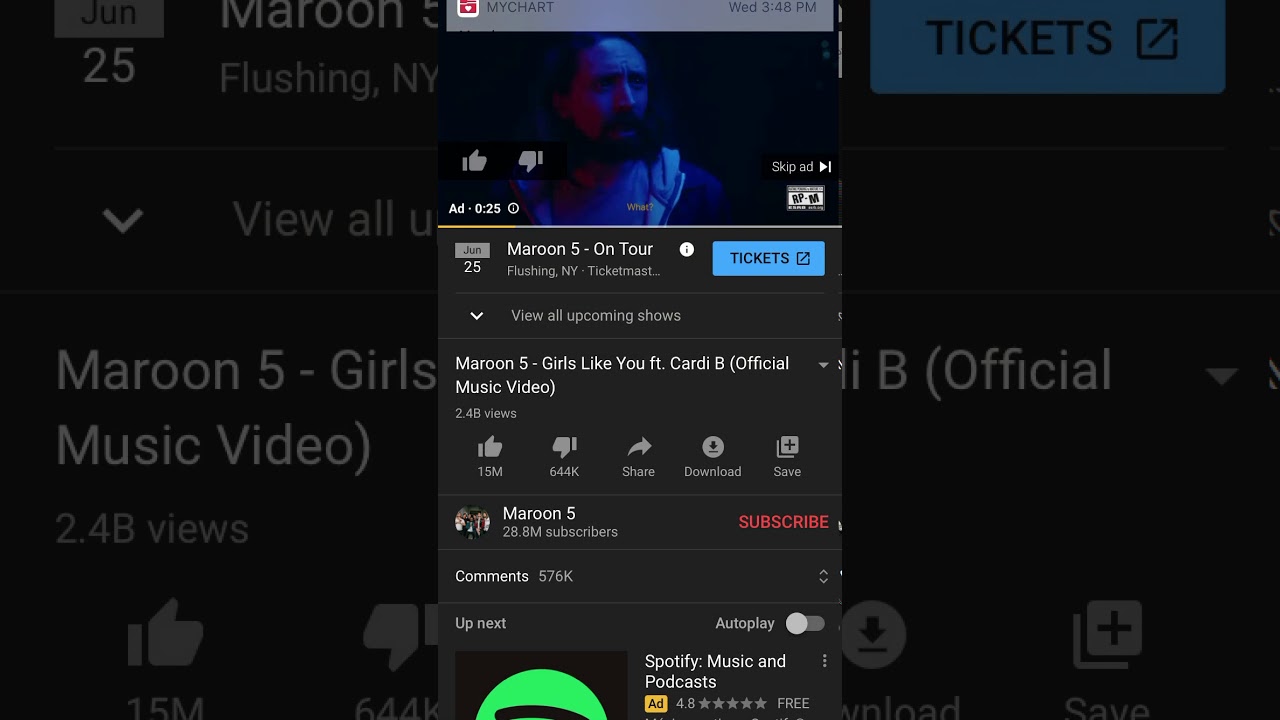The image depicts a dark-themed webpage dedicated to music videos and ticket purchases, specifically focused on the band Maroon 5. At the center of the page, there is a section highlighting a promotional ad featuring a singer from Maroon 5 with options to skip the ad or rate it with thumbs up or thumbs down. 

The ad prominently announces Maroon 5's upcoming tour in Flushing, New York, facilitated by Ticketmaster, with the event scheduled for June 25th. A noticeable blue button is available for users to click and purchase tickets. Below this, there is an option to view all upcoming shows.

Additionally, the page showcases Maroon 5's official music video for "Girls Like You" featuring Cardi B, which has garnered an impressive 2.4 billion views. Engagement metrics are listed, with 15 million likes and 644k dislikes, along with icons for sharing, downloading, and saving the video.

Further down, the band's subscriber count is displayed at 28.8 million, accompanied by a small picture of the group. There is a clickable red "Subscribe" button adjacent to the image. The comments section indicates 576k comments, with an icon allowing users to sort or view them up or down.

Lastly, the "Up Next" section is shown with an autoplay feature that is currently inactive, and an ad for Spotify music and podcasts is visible, boasting a 4.8 rating out of 5 stars, indicating it's available for free.